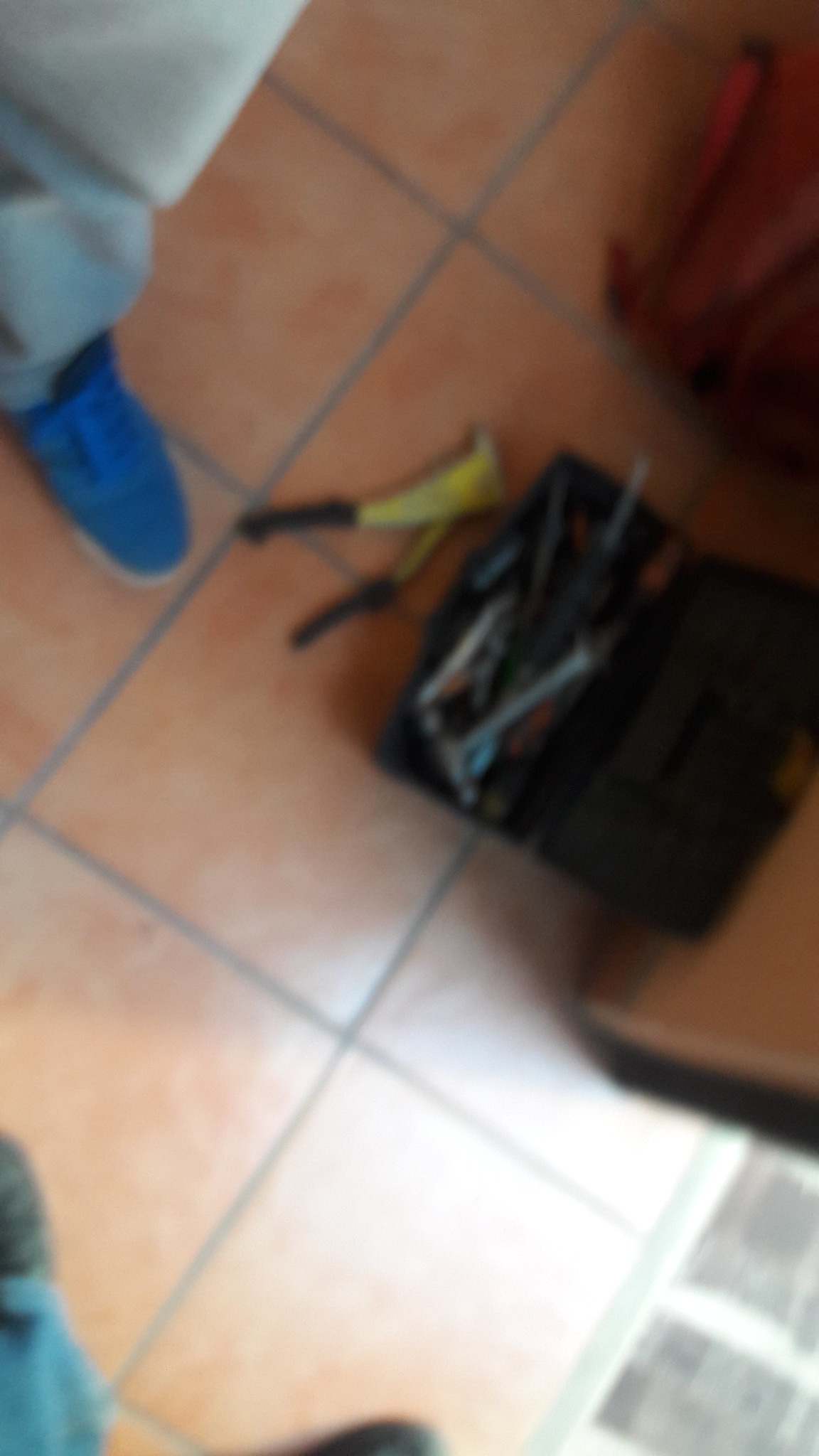This is a blurry color photograph taken indoors, presumably with a head-mounted camera, in narrow portrait mode. The image predominantly features a reddish-brown tiled floor. In the lower left corner, part of a person's left leg and foot are visible. The person is wearing light blue jeans and a blue shoe. Adjacent to this person, there appears to be an open toolbox, overflowing with various tools, including a conspicuous pair of yellow and black pliers laying on the floor. On the extreme right edge of the photo, there's a glimpse of a carpet next to the tiled flooring, illuminated by a light source from the bottom right corner. Part of the photographer's attire is also visible, including a gray shoe and jeans. The top right corner shows a red, indistinct object.